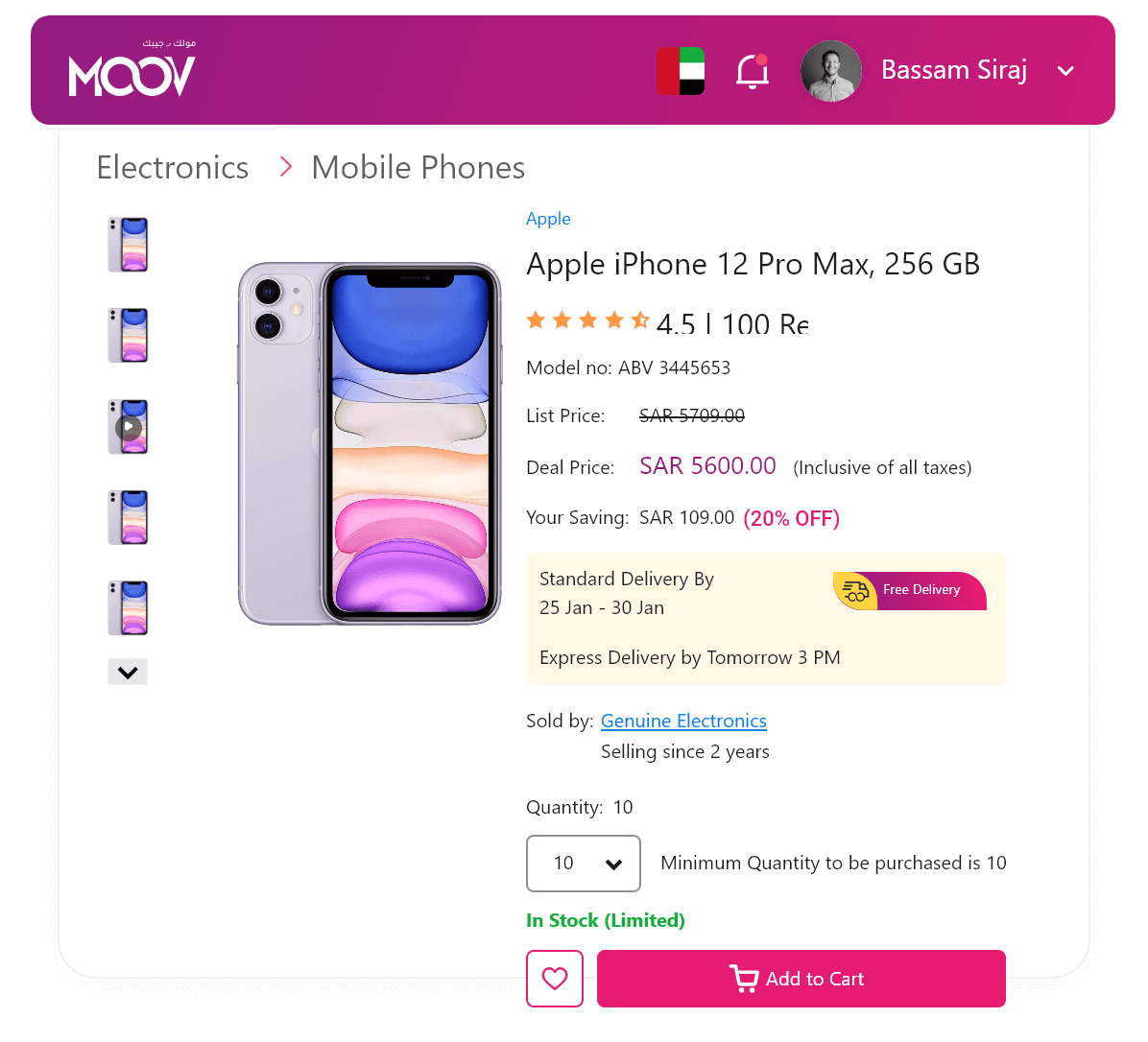The product listing showcases the Apple iPhone 12 Pro Max with 256GB storage. The image on the left features the iPhone itself, while an adjacent pane displays a collection of different iPhone images. The model number is partially visible as "BV" and user ratings indicate a 4.5-star review. The original list price is crossed out. Delivery options include standard delivery by January 25th to 30th, and free expedited delivery by tomorrow at 3 a.m. The seller, Genuine Electronics, has been active for two years. The purchase quantity is set at ten iPhones. There is an "Add to Cart" button as well as a heart icon for wishlisting. The user profile name appears to be Bassam Suraj, though the country selection is unclear. The top of the page features a gradient bar transitioning from pink to purple.